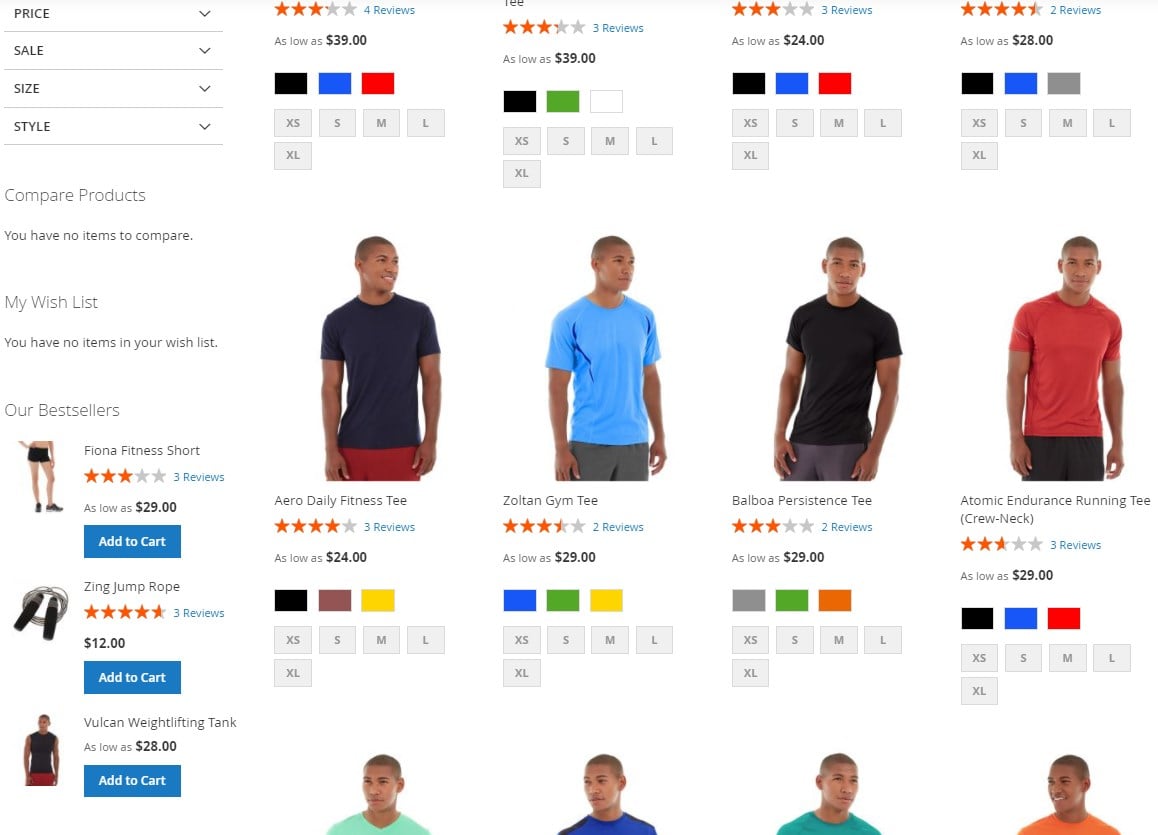This cropped screenshot captures a segment of an apparel website, characterized by a detailed layout of its shopping interface.

In the top-left corner, a portion of a vertical menu is visible, featuring categories like "Price," "Sale," "Size," and "Style," each accompanied by a dropdown box for further selection. Just below this, there's an area labeled "Compare Products," which currently indicates no items selected for comparison. In the central portion of the panel, a section titled "My Wish List" also states that there are no items added to it.

Further down, an "Our Best Sellers" section showcases a vertical list of three featured products. Each product entry includes a thumbnail image on the left, with the product title, customer reviews, price, and an "Add to Cart" button positioned to the right.

To the right of this panel, a grid of t-shirt thumbnails is displayed. Each t-shirt thumbnail is accompanied by a series of small boxes beneath it, representing the available color options for that shirt. Additionally, gray boxes containing sizing letters provide size offerings for each item.

Notably, the very top portion of the image crops out most of the thumbnails, leaving only the number of reviews, price, color options, and sizes partially visible. The second row of t-shirt thumbnails is fully visible, while the bottom row reveals only the upper part of each thumbnail.

This visual presentation provides an organized yet truncated view of the website’s shopping options and product display features.